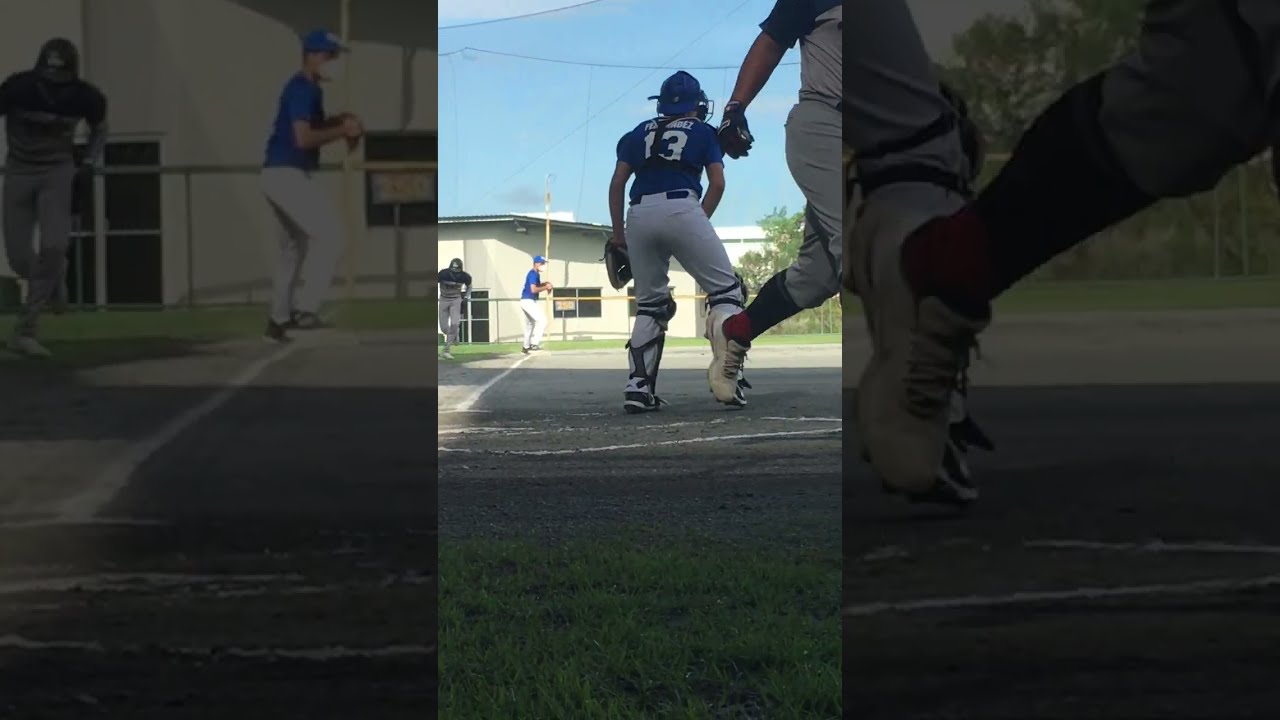In the image, we see a low-angled, behind-home-plate perspective of a baseball game, bathed in sunlight. At the center of the frame, prominently stands the catcher, identifiable by his blue, short-sleeved jersey with the number 13 on it, white pants, and a backward blue cap with a catcher's mask. Positioned just in front of home plate on a patch of green grass, he seems to be anticipating a play. To his left, a runner, clad in a grayish uniform with a blue sleeve, is racing home, seemingly having just rounded third base. Along the third baseline in the background, a white shed-like building and some trees are visible. The right and left sections of the image are shrouded in shadows, but a player’s foot can be seen hitting the ground in the right section, while on the left, the third baseman appears poised to throw. The clear blue sky overhead completes the vivid outdoor scene.